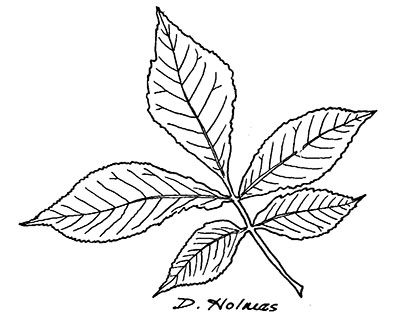This is a simple yet striking black and white line drawing of five pointed leaves attached to a short stem, set against a solid white background. The composition consists of one large leaf at the top, with two smaller leaves on each side below it. Each leaf narrows towards the tip and widens in the middle, featuring detailed black lines indicating the veins. The drawing is minimalist, focusing on the outline and veining of the leaves rather than intricate detail. At the bottom of the image, the artist has signed the piece with the inscription "D. HOL." or possibly "D. Holmes."